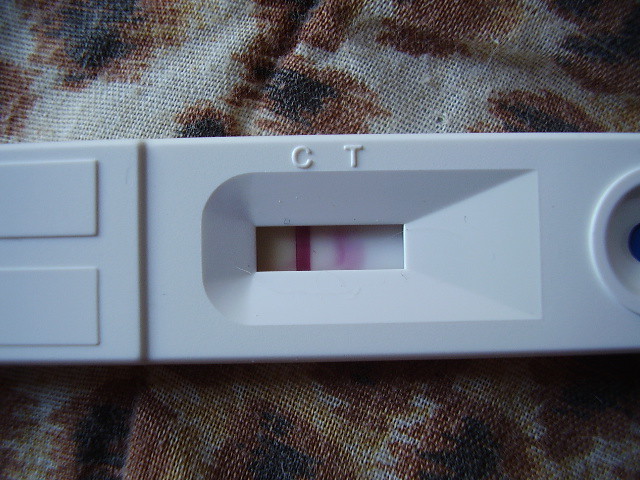The photograph captures a close-up view of a COVID-19 test kit, prominently displayed against a distinctive fabric background adorned with dark brown blotches and even darker brown centers. At the center of the image is an elongated rectangular piece of white plastic, oriented horizontally. The main body of the test features a slightly indented section, marked with the letters "C" (control) and "T" (test), accompanied by a small window showcasing indicator results. A thick red line distinctively marks the "C" position, while a blurry pink line appears at the "T" position. 

On the right side of the test kit, there's a slightly indented circular area designed for placing drops of the sample liquid. On the opposite end, to the left, there's a raised section of the plastic casing featuring two small rectangular elements stacked horizontally. The overall condition of the test suggests a positive result, as indicated by the visible lines in the indicator window.